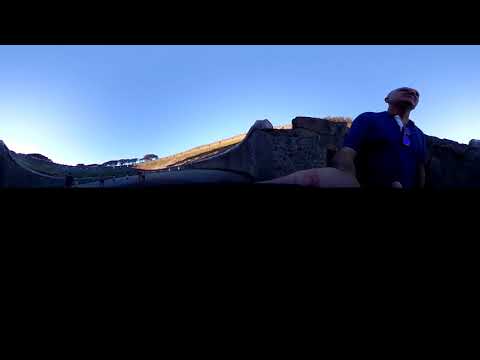This photograph, although of poor quality and distorted, appears to capture a man taking a selfie. A thick, black bar obscures the bottom half of the image, leaving only a narrow two-inch strip visible. The man, wearing a dark polo shirt with sunglasses tucked into the front, extends his arm, likely indicating the use of a selfie stick. His face is raised towards the sky, which is a clear and vibrant blue. The angle of the photograph, taken from a lower vantage point, adds to the distorted effect and shadows, suggesting the sun might be setting. Behind him, a rocky hill formation is visible along with some greenery, possibly trees, indicating an outdoor setting, perhaps during a hike or a walk. Despite the heavy black bars, the remnants of the photograph suggest a serene outdoor scene.